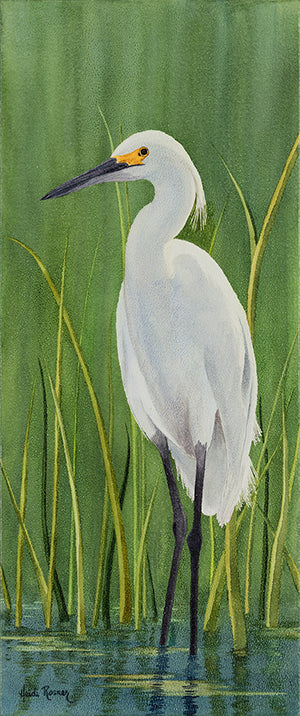This painting depicts a delicate white crane standing gracefully in a marshland, surrounded by blades of grass and blurry water that reflects the sky and background. The bird, facing left, showcases its distinctive features – very long black legs and a slender, black bill that transitions into a bright yellow near the eyes. Atop its head, some white feathers hang loosely. The painting, predominantly vertical and about three times taller than it is wide, is signed in cursive in the lower left-hand corner, possibly by Heidi Rosner, though the signature is somewhat fuzzy and difficult to decipher.